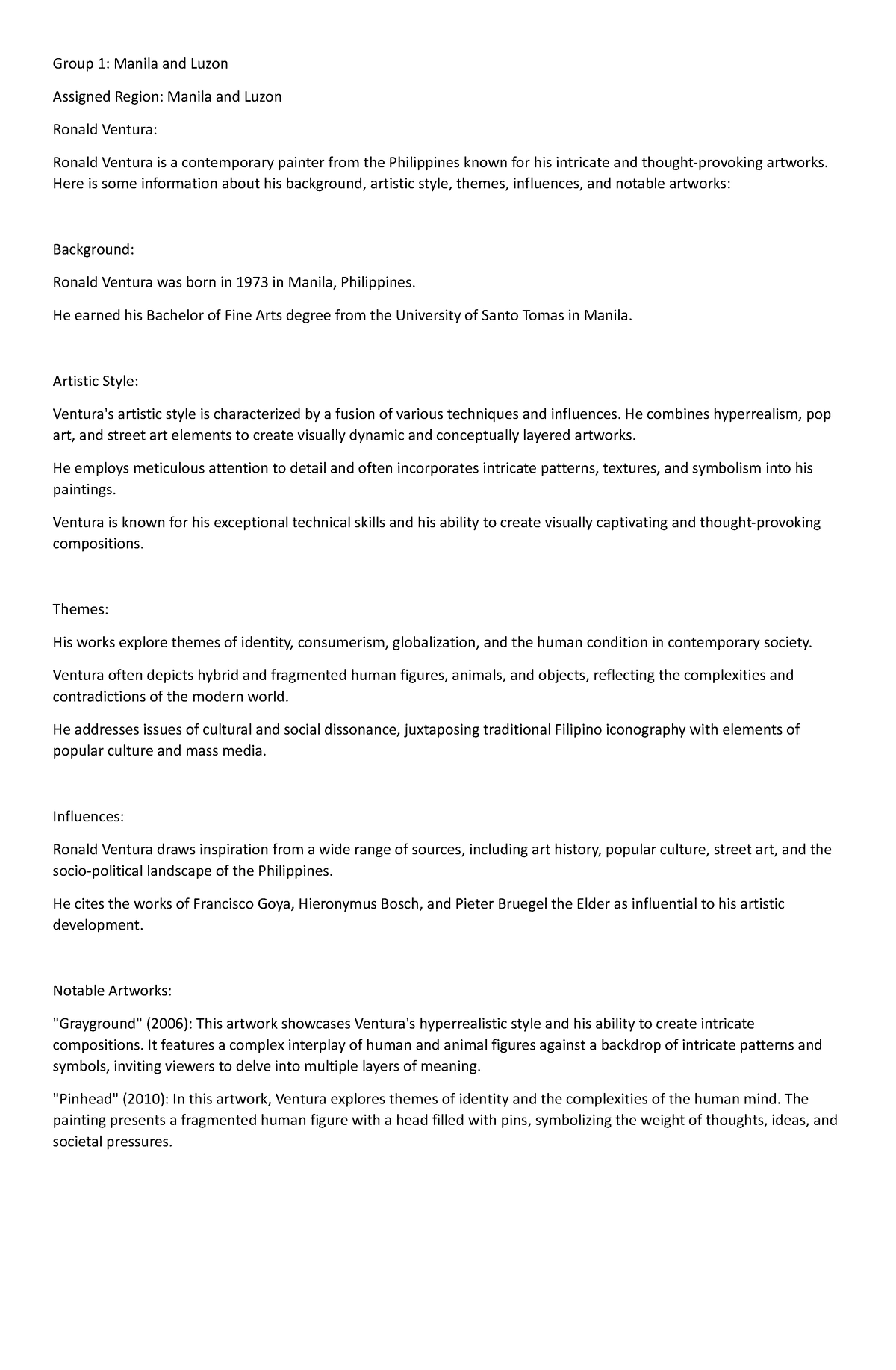"Group 1: Manila and Luzon

Assigned Region: Manila and Luzon
Artist: Ronald Ventura

Ronald Ventura is a contemporary painter from the Philippines, renowned for his intricate and thought-provoking artworks. Born in 1973 in Manila, he earned his Bachelor of Fine Arts degree from the University of Santo Tomas in Manila.

Artistic Style:
Ventura's style is a fusion of hyperrealism, pop art, and street art elements, creating visually dynamic and conceptually layered works. His meticulous attention to detail incorporates intricate patterns, textures, and symbolism, showcasing his exceptional technical skills and ability to craft visually captivating compositions.

Themes:
Ventura's paintings delve into themes of identity, consumerism, globalization, and the human condition in contemporary society. His works often feature hybrid and fragmented human figures, animals, and objects, reflecting the complexities and contradictions of the modern world. He juxtaposes traditional Filipino iconography with elements of popular culture and media to address issues of cultural and social dissonance.

Influences:
Drawing inspiration from a wide array of sources—including art history, pop culture, street art, and the socio-political landscape of the Philippines—Ventura cites artists such as Francisco Goya, Hieronymus Bosch, and Pieter Bruegel the Elder as significant influences on his artistic development.

Notable Artworks:
1. 'Grayground' (2006): This hyper-realistic piece features a complex interplay of human and animal figures set against a backdrop of intricate patterns and symbols, inviting viewers to explore its multiple layers of meaning.
2. 'Pinhead': In this artwork, Ventura explores themes of identity and the complexity of the human mind. The painting depicts a fragmented human figure with a head filled with pins, symbolizing the weight of thoughts, ideas, and societal pressures.

Background: A letter-style format on a white background reads, 'Group 1 Manila and Luzon. Assigned region: Manila and Luzon. Ronald Ventura.' It then provides detailed information about Ronald Ventura's background, artistic style, themes, influences, and notable artworks."